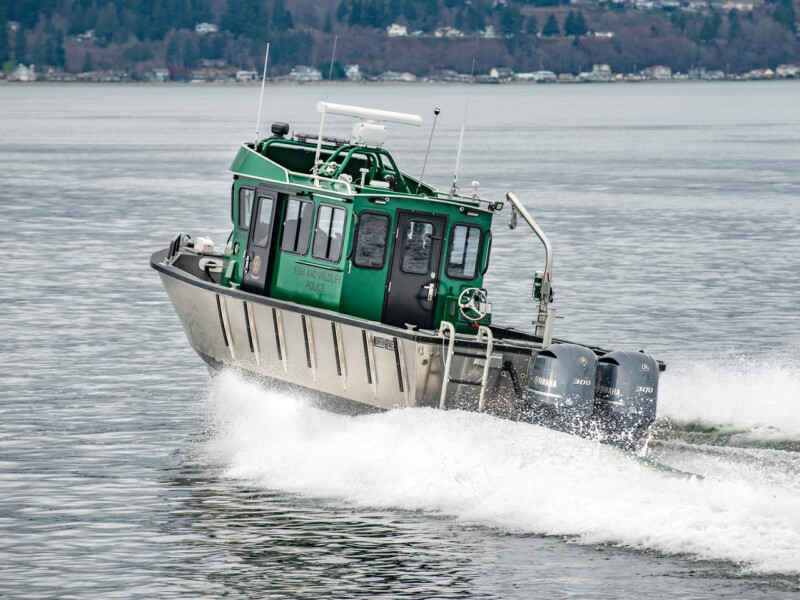The photograph captures a Fish and Wildlife Police lobster boat actively moving through a calm, grey-hued harbor. The boat, which is prominently green with black doors, occupies the center of the image and appears to be moving from the bottom right towards the top left of the frame. It features a deep hull design, with sides that would come up to about three feet if someone were standing inside it. The wellhouse atop the boat is equipped with various antennas and radar equipment. The vessel, boasting a stainless steel trim, is powered by twin outboard motors, each likely delivering at least 100 horsepower, and a white ladder attached to the rear. The boat also has an interior cabin enclosed in glass, as well as an exterior cockpit for steering. Blurred in the distant background are a scatter of homes and businesses along the shore, as well as some indistinguishable boats, indicating a coastal or harbor setting. The water it speeds through just ripples gently, completing the serene yet purposeful scene.